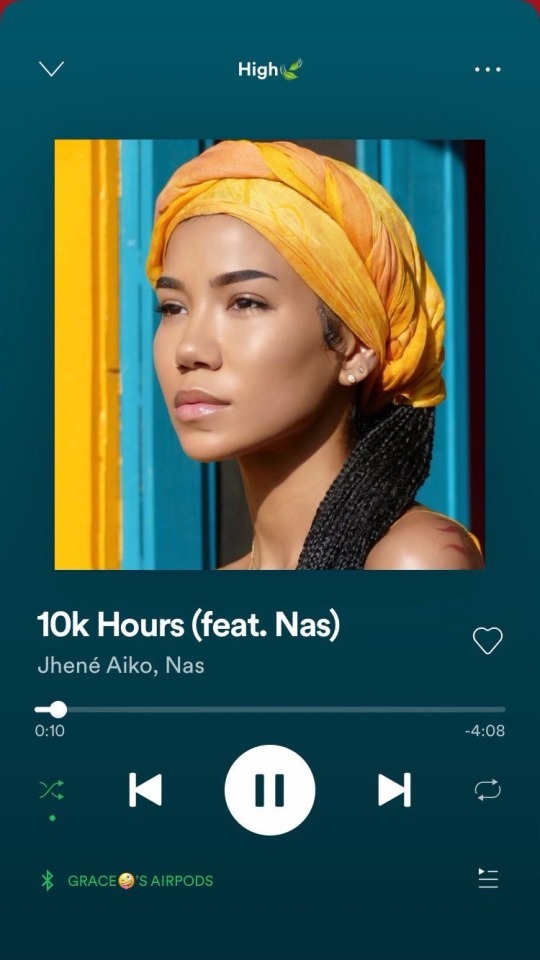The image displays a music app interface with a design reminiscent of Pandora. The background features an inviting aqua-green hue. In the upper left corner, there is a white drop-down arrow, followed by the word "Hi" in white with a capital "H" and an adjacent symbol resembling two bean sprouts. On the upper right corner of the screen, there are three white horizontal dots indicating additional options.

The central focus of the image is a female artist, depicted with black hair and a whitish-yellowish scarf elegantly draped over her head, gazing thoughtfully toward the left side of the screen. Below her portrait, the text "10K Hours featuring Nas" is prominently displayed in white, indicating the current song. The playback progress bar shows that the song is at the 10-second mark, with a total duration of 4 minutes and 18 seconds.